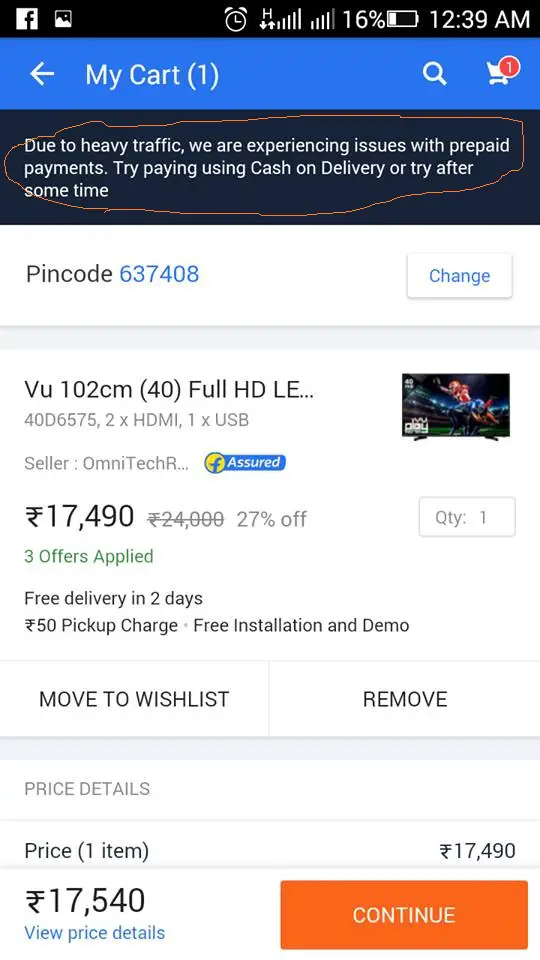**Detailed Caption:**

This screen capture depicts a user's mobile shopping cart on an unidentified website, characterized by a light blue header bar at the top. The text in the header reads "My Cart" and indicates "1 item" in the cart. Directly below this, a dark blue notification bar alerts users about issues with prepaid payments due to heavy traffic, suggesting alternatives such as cash on delivery or trying again later. This notification is emphasized with an orange jagged circle, drawing attention to the message.

Below the notification, the pin code for the delivery area is displayed. The main section features a summary of the cart's contents, including a small image of the item, the seller's name, price, delivery details, and quantity. There are also options to move the item to the wishlist or remove it from the cart.

Further down are additional pricing details, with a prominent orange "Continue" button at the bottom of the screen to proceed with the checkout process.